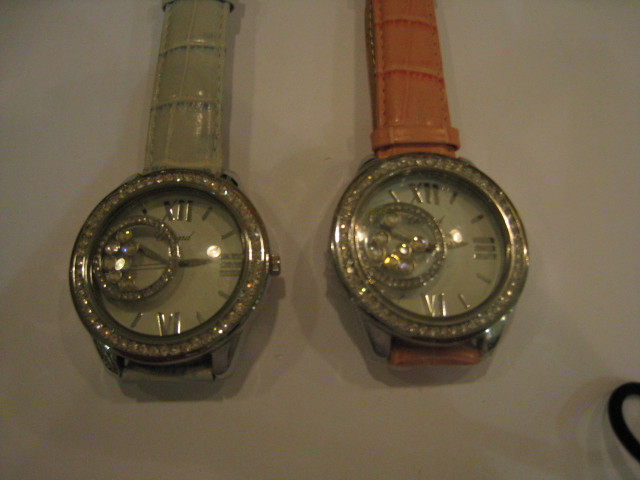This image features two elegant wristwatches displayed side by side. Both watches are identical except for the colors of their bands; the watch on the left sports a light blue leather band, while the one on the right has a light pink leather band. The faces on both timepieces are pristine white, adorned with shimmering rhinestone frames that form a circular shape around the edge. The watch faces are detailed with Roman numerals and silver lines, with the hands also crafted in silver for a sophisticated touch. Additionally, each watch has a smaller inner circle on its face, surrounded by another ring of rhinestones, and filled with what appear to be other small crystals or gemstones. The background is a clean, white surface, providing a neutral backdrop that highlights the refined details and colors of the wristwatches.